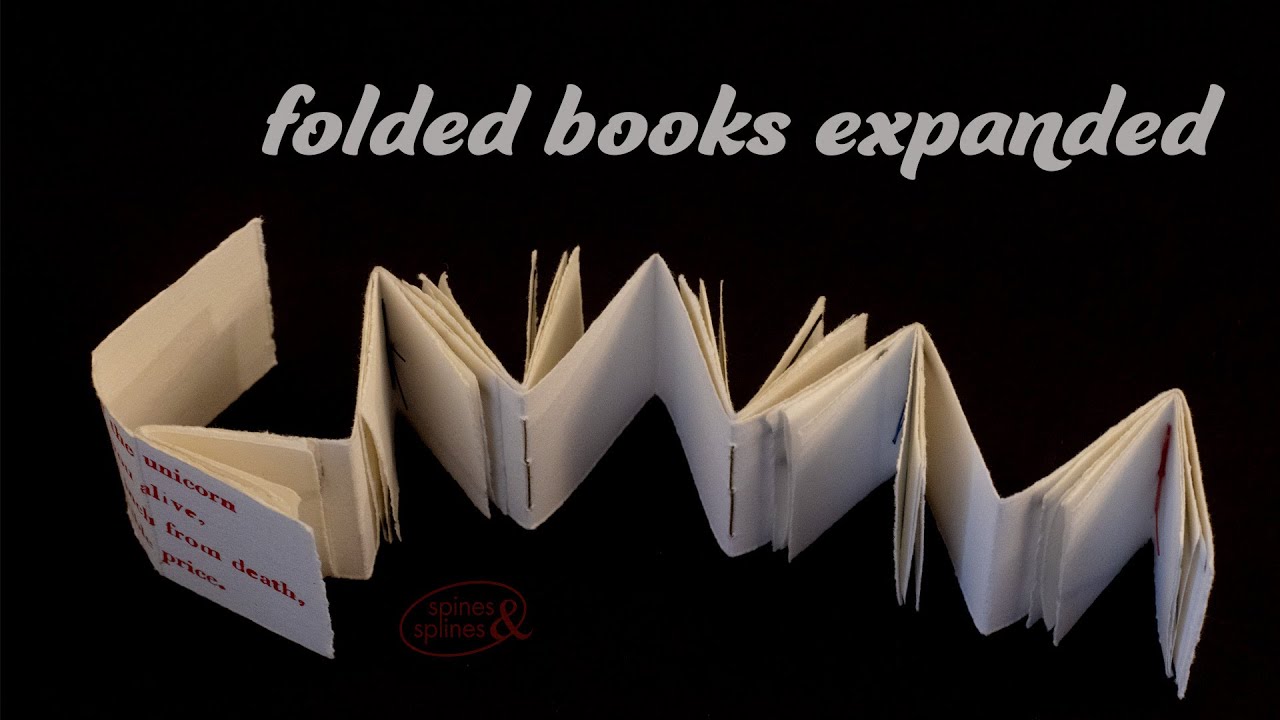The image features a striking poster with a black background and light gray text at the top that reads "Folded Books Expanded." Dominating the poster is a series of white paper pages, intricately folded in an accordion style, creating a pattern of upright book fragments that extend horizontally across the image. The paper, appearing rough and possibly handmade, is bound tightly with visible stitches, lending an artisanal feel. On the leftmost page, red text stands out, fragmentarily displaying the words "Unicorn," "Alive," "From Death," and "Price." Below the folded paper arrangement, in almost barely noticeable red lettering, is an emblem for "Spines and Spines," further suggesting a connection to a bookbinding or literary-themed company. The composition and layout evoke a sense of depth and complexity, inviting viewers to ponder the tactile and visual experience of expanded, foldable books against a stark, black backdrop.